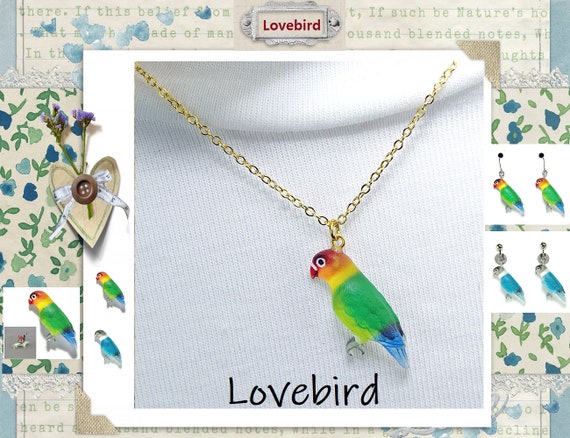This is a detailed advertisement for "Lovebird" jewelry, featuring a colorful and imaginative parrot-themed design. The centerpiece is a gold chain necklace with a pendant of a vibrant parrot. The parrot has a red beak, red head, orange and yellow cheeks, a yellow neck, a light green stomach with green feathers, and an indigo-to-blue tail. The background includes a white shirt, suggesting the necklace being worn. The top of the ad prominently displays "Lovebird" in black text.

To the left of the main image, there's a close-up of the pendant. The right side showcases additional options, including earrings featuring the same parrot design. Alongside, there are blue-colored parrot earrings with a white head. The border is adorned with mosaic-like elements, with blue and light green flowers, creating an aesthetically pleasing frame. The overall design includes typewriter-style passages, watercolor effects, and pastel elements, enhancing the ad's artistic appeal. This visually rich ad emphasizes the "Lovebird" collection of parrot-themed jewelry, presenting various colorful options for potential buyers.